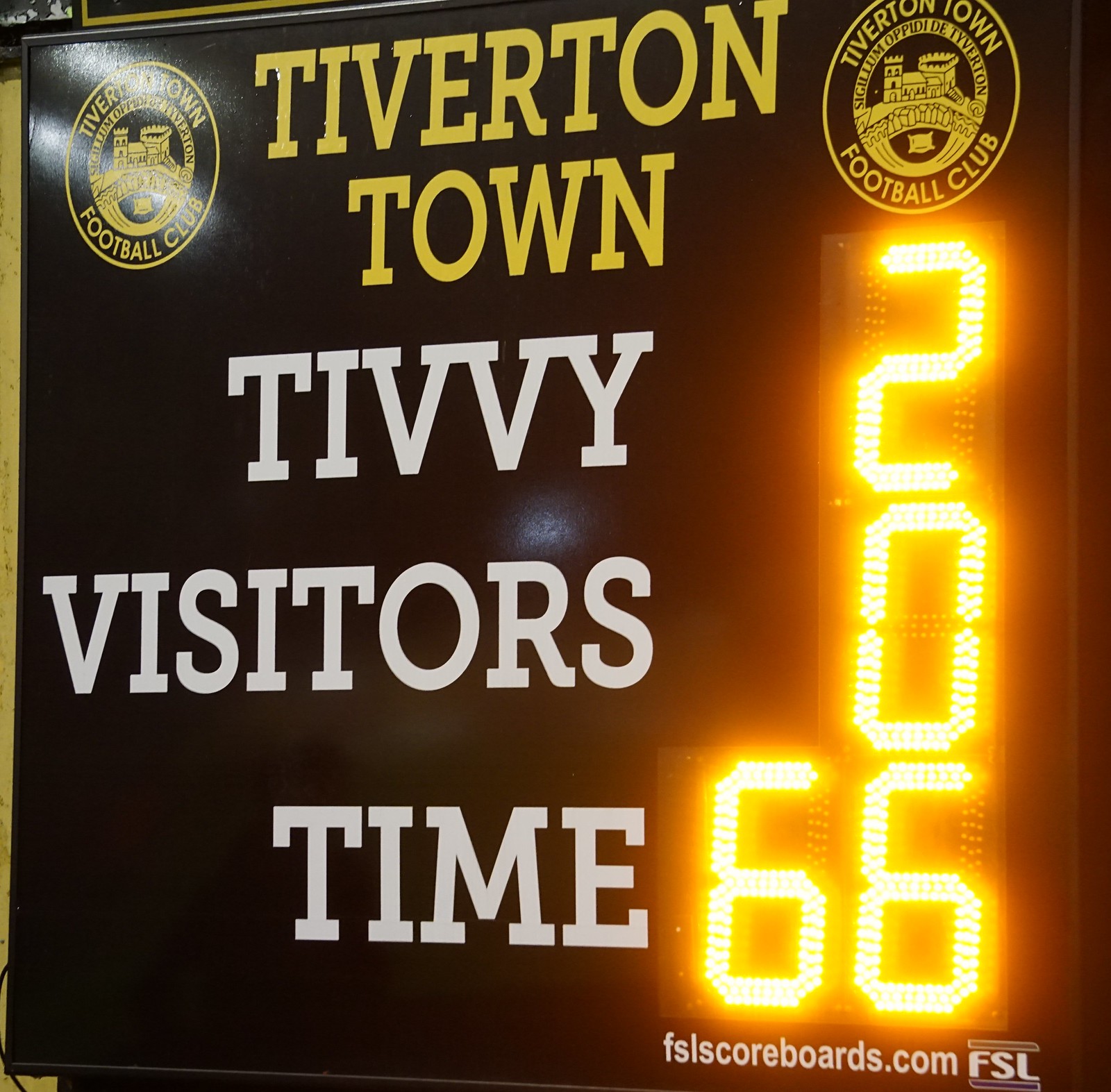The image is a close-up of the scoreboard for Tiverton Town Football Club, with a detailed design and illuminated display. The background of the scoreboard is black, while the overall framework has a brown tone. At the top, in large, bold, gold letters, it reads "Tiverton Town," and directly below, in white letters, it spells out "T-I-V-V-Y." The logo of Tiverton Town Football Club is prominently featured twice: once at the top and again to the right of the main text. This logo consists of a gold circle within another gold circle against a black background, featuring a drawing that resembles a castle or fort and a wall. Below "T-I-V-V-Y," the scoreboard displays "visitors" in white text, followed by "time." The LED panel shows the current score, with "2" for Tivy, "0" for visitors, and the time "66" illuminated in yellow. At the very bottom, the URL "FSLScoreboards.com" is displayed in small white text, along with the abbreviation "FSL."